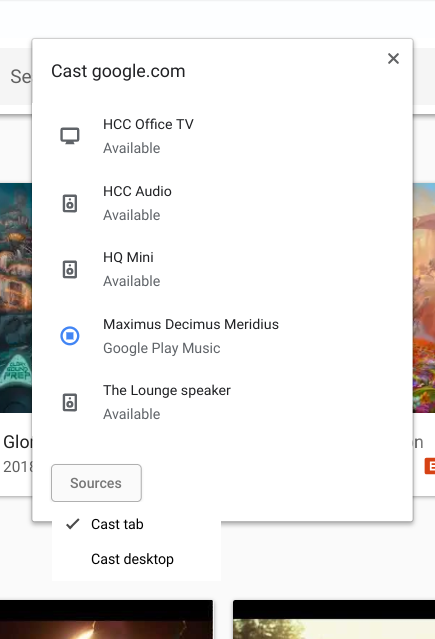A screenshot of a webpage from castgoogle.com is displayed, featuring a white rectangular pop-up box in the center. The pop-up box lists available casting devices with the heading "castgoogle.com" (where "cast" is capitalized and "google.com" is lowercase). On the top-right corner of the pop-up, there is a cancel icon resembling an 'X'.

Within the pop-up box, the first section showcases a computer monitor labeled "8cc office TV" with an "available" status. Following that, there's a speaker labeled "8cc audio" marked as available. Another speaker icon is listed with the label "HQ Mini," both words capitalized, indicating its availability.

Beneath the devices, the box lists "Maximus Decimus Meridius" twice, suggesting it is the current media being played, accompanied by a blue stop icon. The text "Google Play Music" below this indicates the source of the audio. Further down, another speaker labeled "lounge speaker" is marked as available, with a speaker icon to the left of the label.

At the bottom, there are two options under "sources": "Cast tab" and "Cast desktop," with the "Cast tab" option currently selected.

Below the pop-up box, an image of a movie cover is partially visible, but the focus remains on the detailed options available for casting media through the interface.